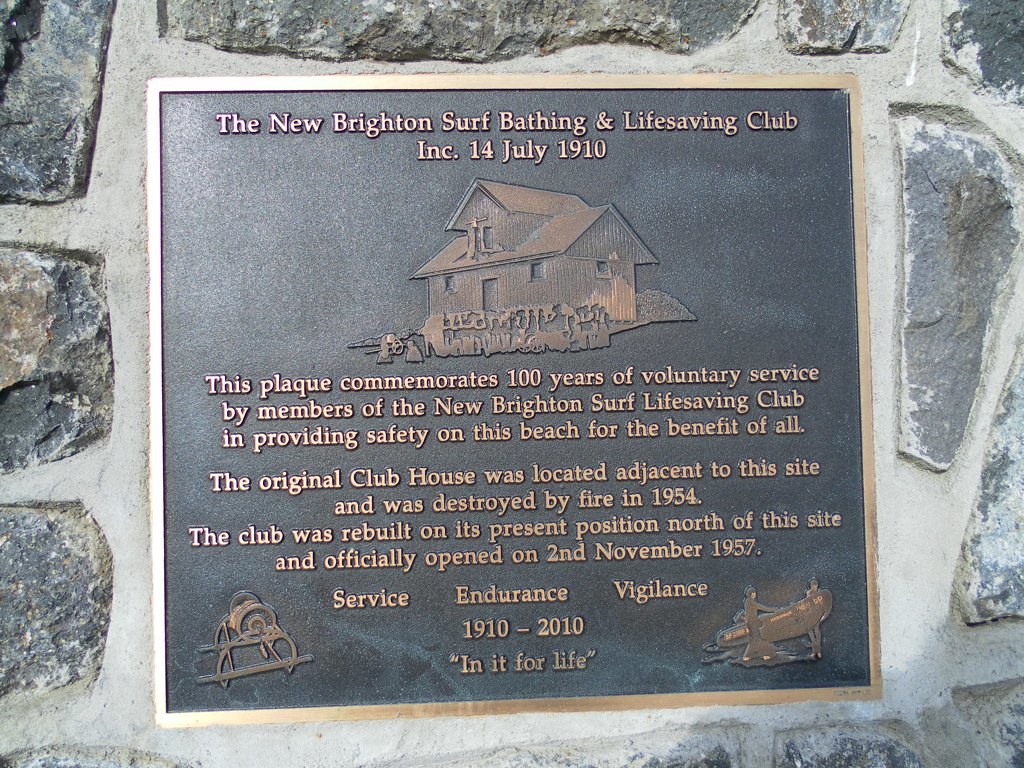This detailed color photograph, in landscape orientation, captures a commemorative bronze plaque with gold lettering and a gold frame embedded into a stone wall. The plaque stands out against the individually cemented stones, its headlined text reading, "The New Brighton Surf, Bathing, and Life-Saving Club, Inc., 14 July 1910." Below the headline, an illustration depicts a small wooden building with a gable roof, evocative of the original clubhouse. The plaque's main body of text solemnly commemorates "100 years of voluntary service by members of the New Brighton Surf Life-Saving Club in providing safety on this beach for the benefit of all." It recounts that the original clubhouse, once adjacent to this very site, was tragically destroyed by fire in 1954. Rising from the ashes, the club was rebuilt at its current location north of this site and officially reopened on 2 November 1957. The values "Service, Endurance, Vigilance" prominently mark the passage of a century from 1910 to 2010, concluding with the heartfelt motto, "In it for life." Intricate engravings adorn the bottom corners of the plaque: a cannon on the left and an airplane on the right, adding to the historical and representational realism of this significant memorial.